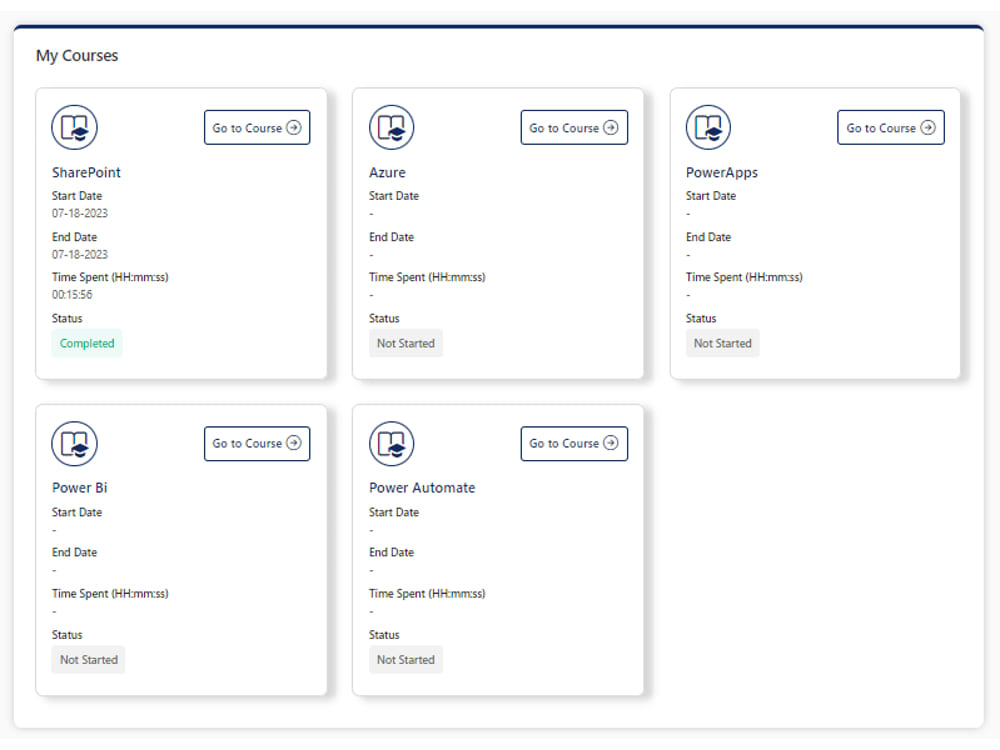The image depicts a white screen with a thin blue line at the top. Below this line, the header reads "My Courses," accompanied by a book icon. Each course entry is similarly formatted with a "Go to course" button featuring a right-pointing arrow. The courses listed are as follows:

1. **SharePoint:**
   - **Start Date:** 07/18/2023
   - **End Date:** 07/18/2023
   - **Time Spent:** 3 hours, 15 minutes, 56 seconds
   - **Status:** Completed

2. **Azure:**
   - **Start Date:** —
   - **End Date:** —
   - **Time Spent:** —
   - **Status:** Not Started

3. **Power Apps:**
   - **Start Date:** —
   - **End Date:** —
   - **Time Spent:** —
   - **Status:** Not Started

4. **Power BI:**
   - **Start Date:** —
   - **End Date:** —
   - **Time Spent:** —
   - **Status:** Not Started

5. **Power Automate:**
   - **Start Date:** —
   - **End Date:** —
   - **Time Spent:** —
   - **Status:** Not Started

In each course entry, the book icon is shown inside a blue circle, and the respective course names are highlighted in blue text.